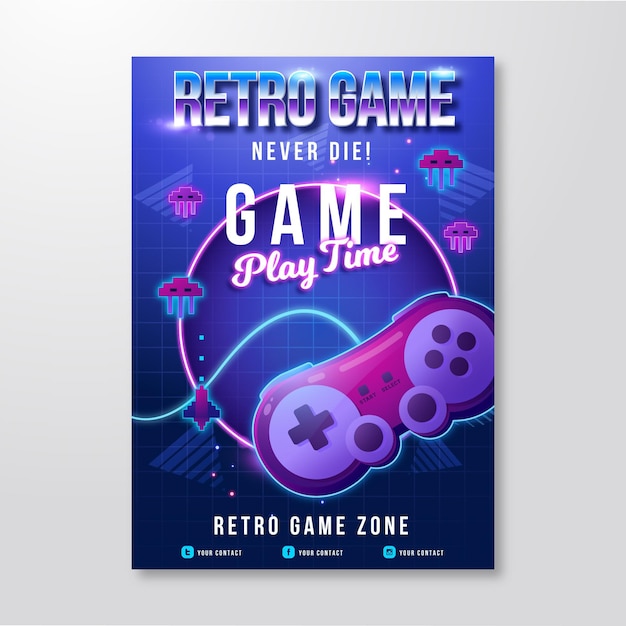The image showcases a vibrant and nostalgic design reminiscent of old movie posters or classic video game advertisements. Dominated by a purplish-blue background that transitions to a lighter shade towards the top, it prominently features the text "Retro Game" in half blue, half purple text at the top, followed by "Never Die" in striking white text. Centrally, a large neon pink circle takes the spotlight with the words "Game Playtime" inscribed at the top. Surrounding the circle are four asteroid-like or squid-like characters, evoking a sense of classic arcade games, possibly reminiscent of Pac-Man ghosts. At the bottom right of the circle, there's a distinctive game controller in pink and purple, adding a touch of retro gaming charm. At the very bottom of the image, "Retro Game Zone" is boldly displayed, while "Your Contact" is repeated three times in a smaller font. The overall color palette includes various shades of pink, blue, red, and purple, enhancing its retro aesthetic.